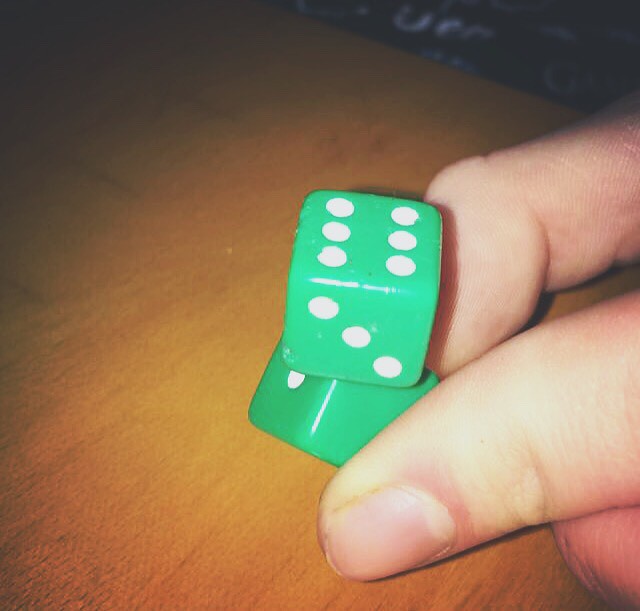The photograph presents a close-up scene featuring a pair of green dice held between the thumb and index finger of a Caucasian individual. The dice are positioned over a wooden tabletop with a distinctive texture, possibly vinyl-like with a light tone, darkened at the corners as though a filter has been applied. The top die prominently displays three white dots on the side facing the camera and six white dots on its top surface, while the bottom die reveals a blank green face with a single white dot on the left-hand side visible. The hand holding the dice is illuminated from above, casting a bright shine on the dice and creating a circular light reflection on the table, while the surrounding area falls into dark shadows. The person's fingernails are noticeably short but carry visible dirt, adding a gritty element to the otherwise methodical composition. In the background, a black cloth drapes down from the upper right corner, contrasting with the lighter tones of the table and bringing depth to the image.